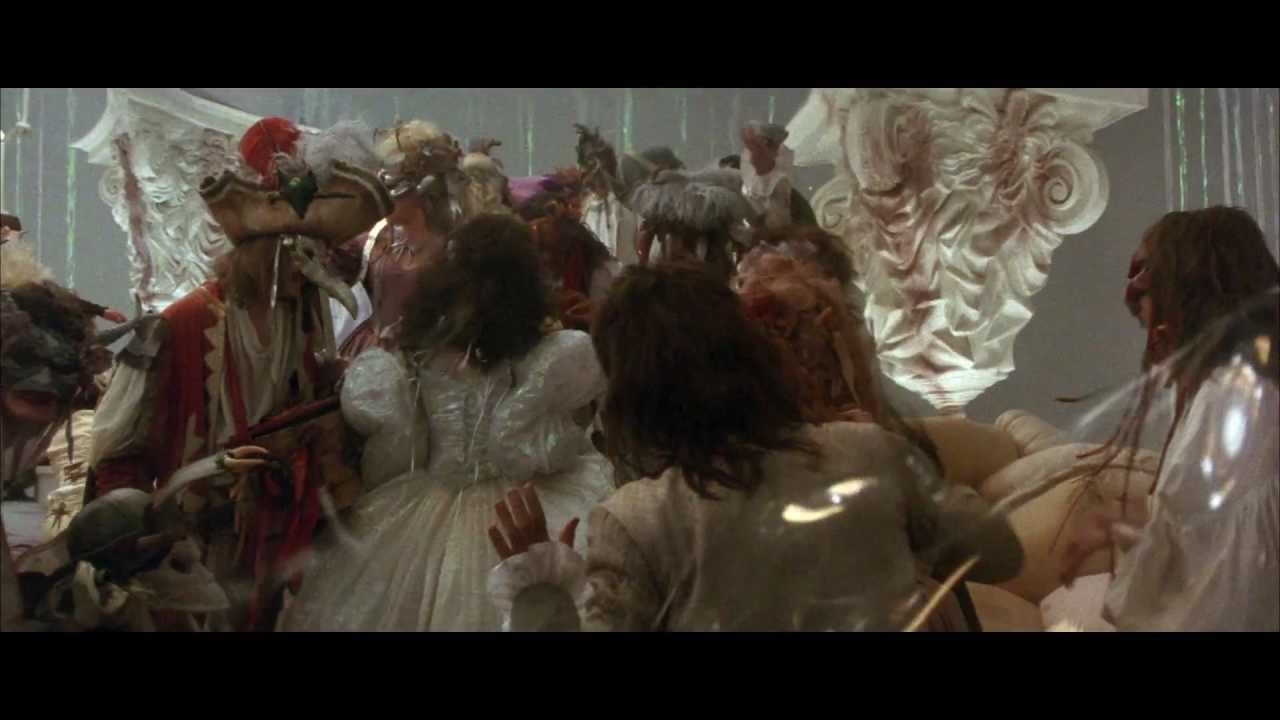This image is a detailed widescreen still from a film set in a period reminiscent of Marie Antoinette's era, portraying a chaotic masquerade scene. The frame is flanked by black bars on the top and bottom, accentuating its cinematic format. At the heart of the image, amidst muted tones, a lively and somewhat tumultuous party unfolds. The central figure is a woman adorned in a voluminous white Victorian dress with poofy shoulders and curly hair. To her left stands a man in a large pirate hat and a beak mask, while numerous other characters, mostly Caucasian, don elaborate masks and fanciful Renaissance attire in shades of white, gray, and beige. The atmosphere, though festive, hints at violence, with splashes of a red substance resembling blood on ornamental white marble statues in the background and on several participants. The scene blends elements of elegance and chaos, suggesting a bohemian yet disturbed social gathering.